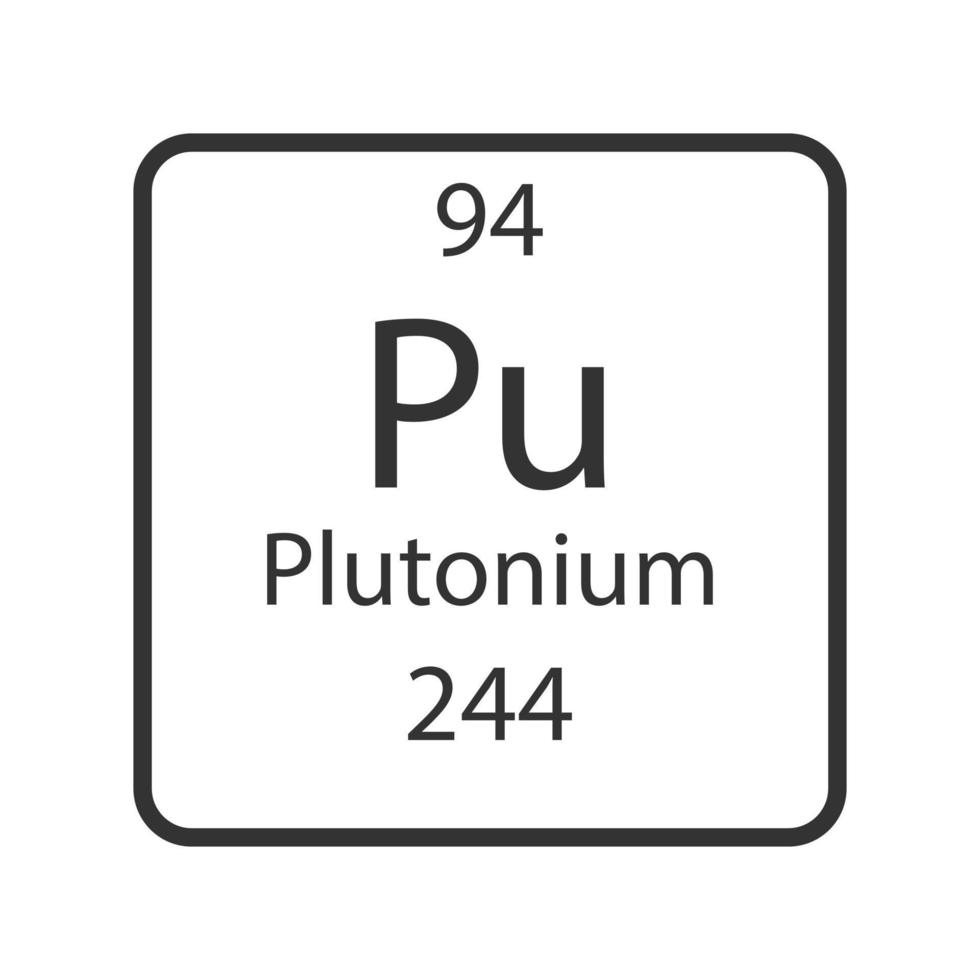The image depicts a rectangular card representing the element Plutonium from the periodic table, set against a white background. The card itself is white with a prominent black border that features slightly curved corners. At the top of the card is the number "94," which denotes the atomic number of Plutonium. Below this number are the letters "Pu," with the "P" capitalized and the "u" in lowercase, displayed in the largest text on the card. Underneath "Pu" is the word "plutonium," followed by the number "244," indicating its atomic mass. The overall design is minimalistic, suggesting that this card is a part of a larger periodic table.